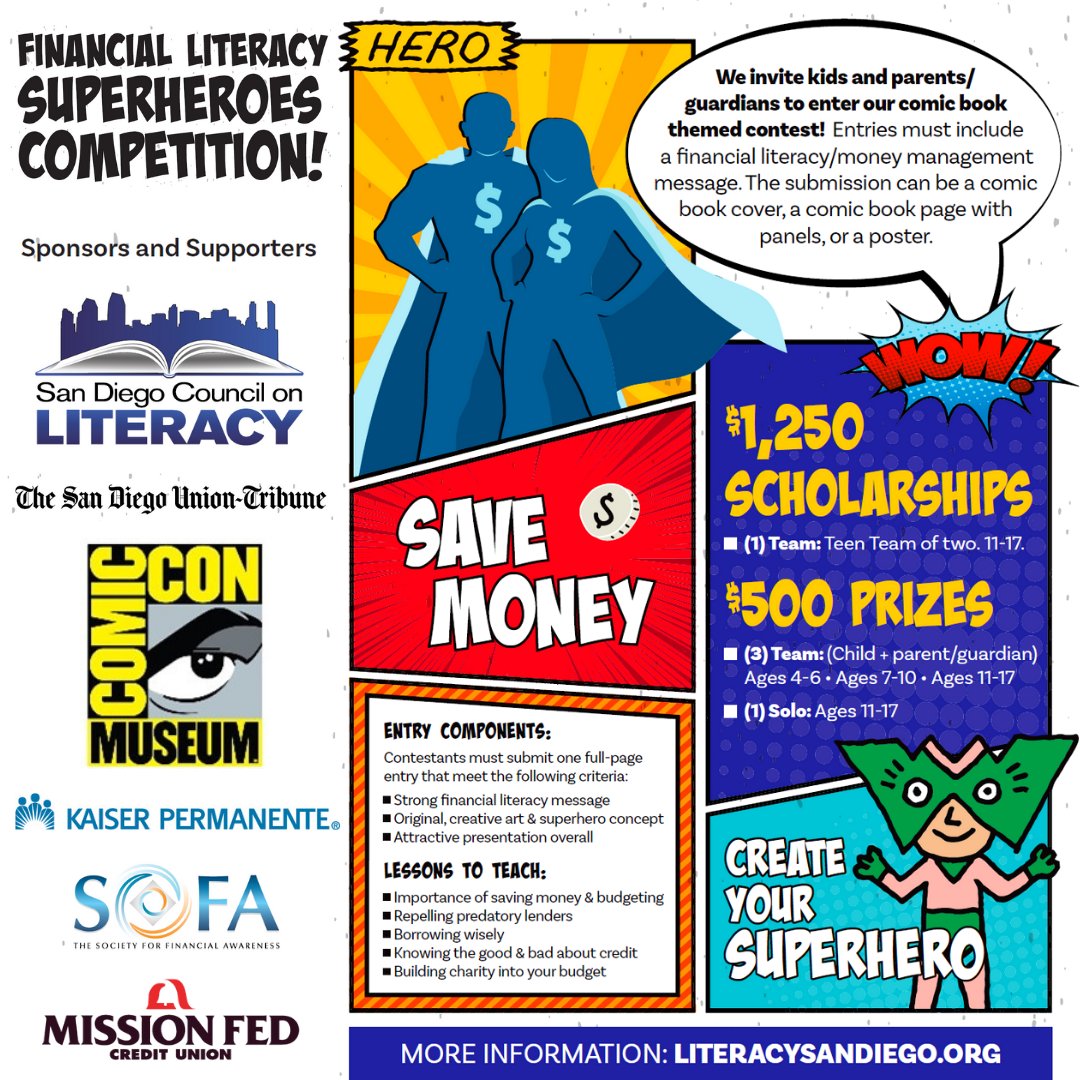This poster, in a vibrant comic book style on a white background, promotes the San Diego Council on Literacy's Financial Literacy Superheroes Competition. The headline, "Financial Literacy Superheroes Competition," is prominently displayed in black lettering, inviting kids, parents, and guardians to participate. Through the comic book theme, entries must deliver a financial literacy or money management message and can be submitted as a comic book cover, a comic book page with panels, or a poster.

The left side of the poster lists all the sponsors and supporters, including the San Diego Union-Tribune, Comic-Con Museum with its iconic yellow, black, and gray logo, Kaiser Permanente, Mission Federal Credit Union, and SOFA, a San Francisco-based organization. A city line graphic with an open book in front adds a creative visual element.

Key contest details include offering a $1,250 scholarship to the top teen team (ages 11-17), and additional $500 prizes for teams comprising a child and a parent or guardian across different age groups: ages 4-6, 7-10, and 11-17. There's also a solo prize for ages 11-17. The poster features comic book-style lettering such as "WOW!" and encourages participants to "Save Money." At the bottom, a small superhero character with a green mask, pants, and gloves prompts viewers to "Create Your Superhero." For more information, it directs to literacysandiego.org.